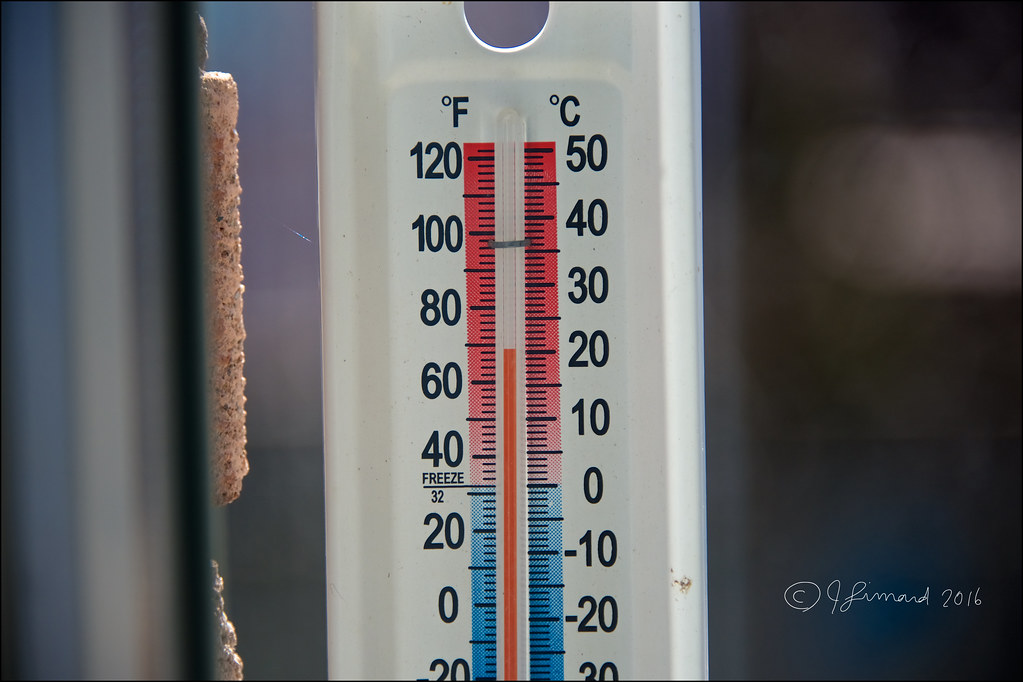In the center of the image, there is a horizontally-oriented, rectangular device prominently displayed. This device covers the central portion of the image entirely. The top part of the device features a cutout, slightly obscured by the photo's framing, revealing a glass tube thermometer inside. On the right side of the device, there are markings indicating temperatures in degrees Celsius, labeled with numbers descending from 50 at the top, through 40, 30, 20, 10, 0, and continuing into the negative range with -10, -20, and -30 at the bottom. 

On the left side, the thermometer shows temperatures in degrees Fahrenheit, with increments labeled from 120 at the top, followed by 80, 60, 40, a midpoint at 32, then descending to 20, 0, and -20. The temperature scale is color-coded: red from 0°C upwards and blue from 0°C downwards, and similarly red from 20°F upwards and blue from 20°F downwards.

In the lower right corner of the device, there is a copyright symbol (©), followed by the text "I. Fehmarn 2016," written in white. The background of the image is blurry, with a clear view of a brick wall on the left. The wall is composed of brown bricks with a notable stone on the edge, adding texture to the otherwise hazy backdrop.